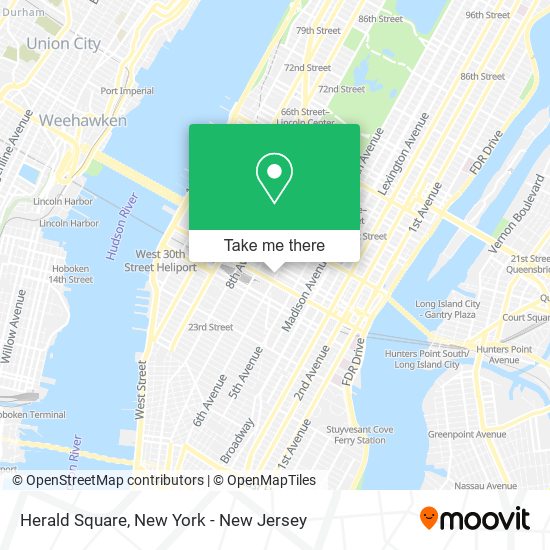This image is a detailed screenshot of the MOOVIT (spelled M-O-O-V-I-T) application map, showcasing its user interface and map features. To the left of the lowercase "moovit" text is a small, smiley face map pin icon. The main portion of the image is dominated by a map of New York, specifically focusing on the Long Island area. 

Overlaying the map is a floating photograph with the text "Take me there," indicating an option to initiate navigation to the highlighted location. The map reveals a complex network of streets and landmarks, including significant intersections and a street that cuts through at an unusual angle. Notably, the map resembles Google Maps but is distinguished by the presence of credits at the lower-left corner, which include "OpenStreetMap Contributors" and "OpenMapTiles."

Prominent landmarks and streets are visible, such as Herald Square, the Hudson River, and various significant streets like 86th Street, Madison Avenue, 5th Avenue, Broadway, FDR Drive, and Vermont Boulevard. The map also displays major infrastructure elements like bridges, wharfs, and subway lines that traverse under the water, highlighting the comprehensive nature of the mapping.

This descriptive screenshot offers a thorough overview of the spatial layout and key features in this New York and Long Island region, enhanced by detailed map tiles and the useful "Take me there" navigation option.